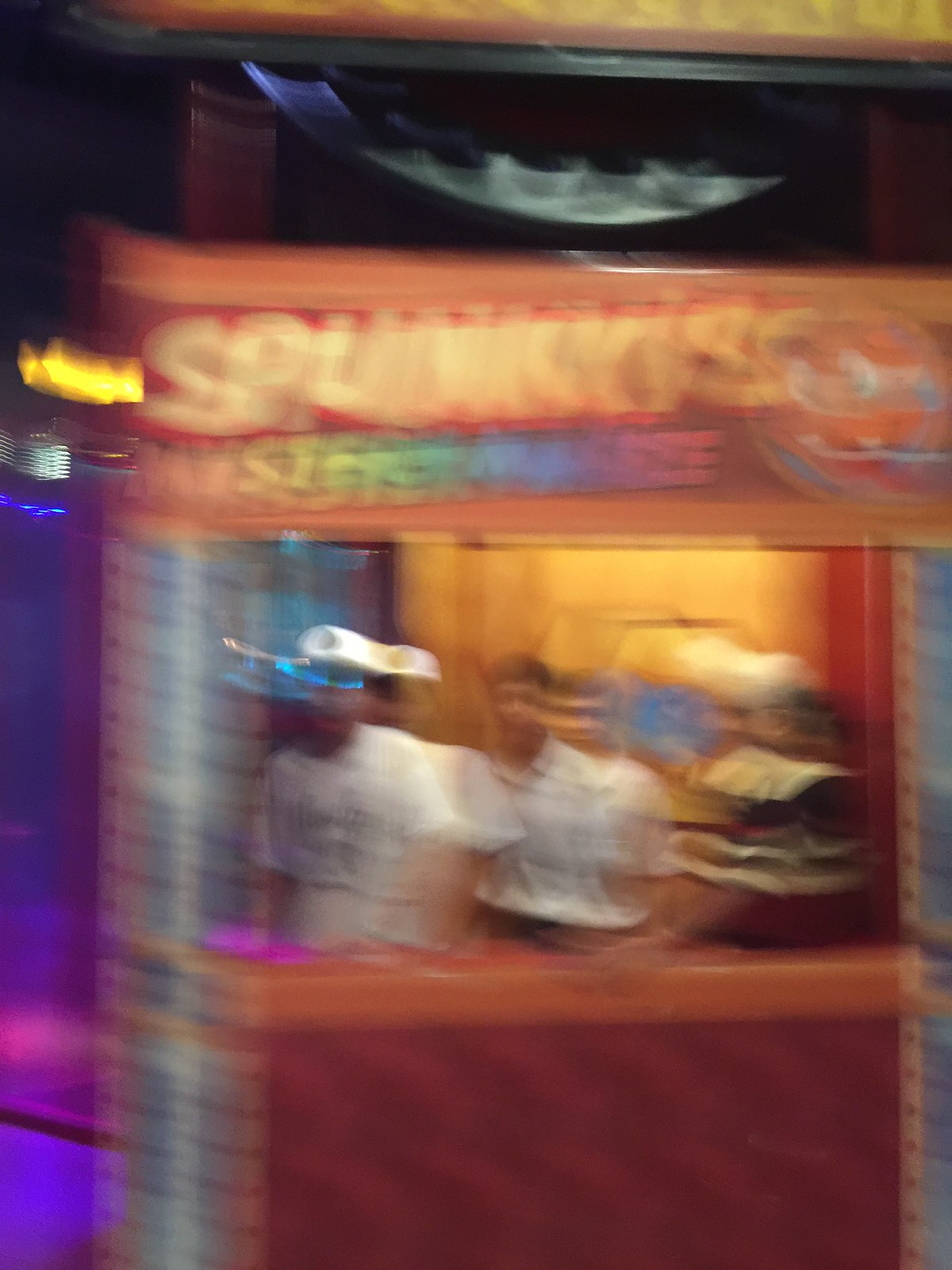This image is a blurry color photograph taken outside at night, possibly at a to-go style restaurant or booth. The vibrant and bright colors set against the dark background create a strong contrast. The front of the booth is red with an orange counter, and the sides have barber pole-style metal sections. Despite the blur, there are three people standing behind the counter, all wearing white shirts, and one appears to be wearing a white hat. Above the booth is a sign with graffiti-style writing, which could spell "Spelunkies" and possibly includes a one-eyed red ogre or goblin face next to the text "mystery maze" in rainbow coloring. A blurry object above the sign might resemble a bat or poltergeist. The photograph appears to have been taken with the camera moving diagonally from the top portion to the center, and there's an overall sense of motion and lack of focus, contributing to the image's indistinct and chaotic appearance.